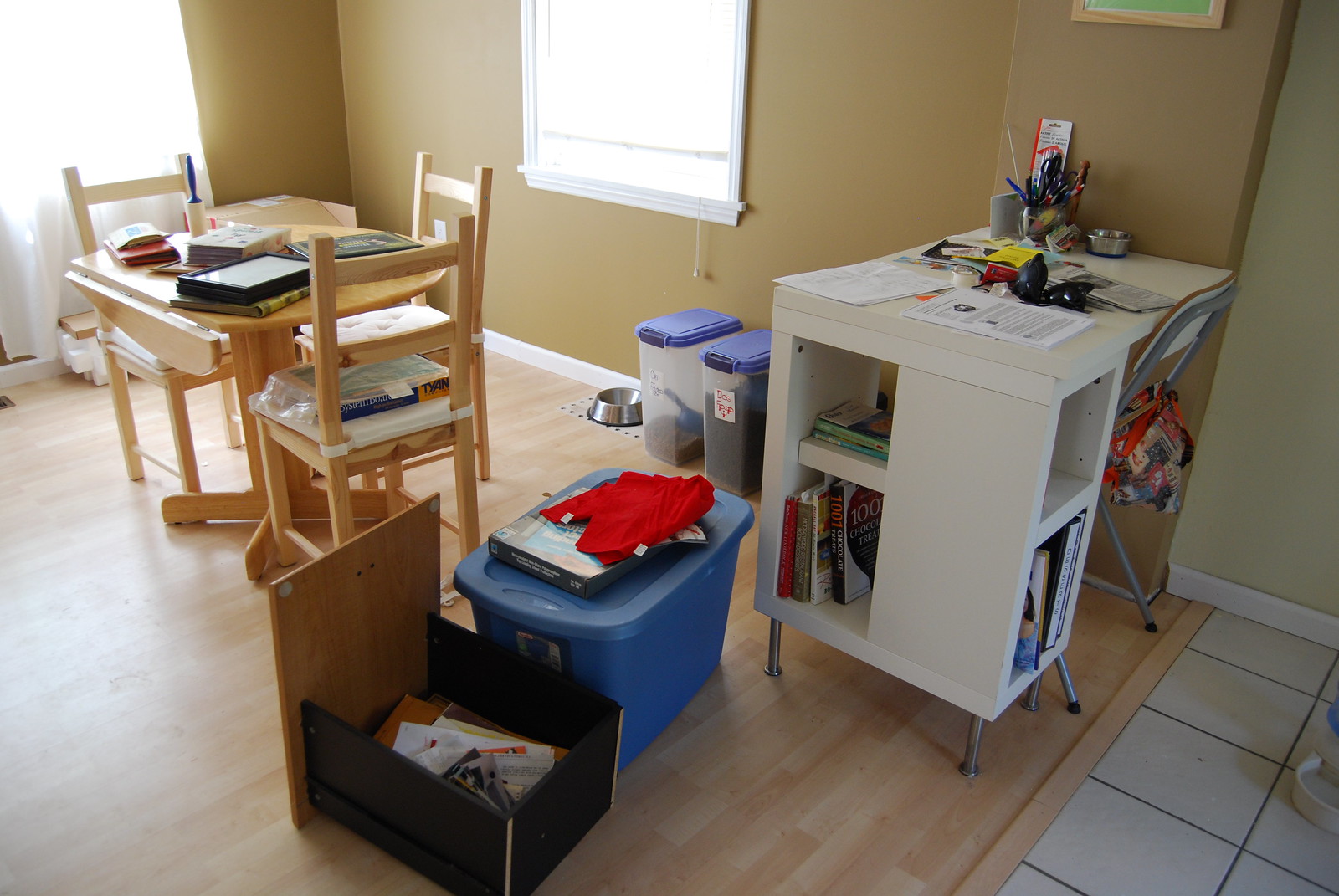The image depicts a dining room that is part of a combined kitchen-dining area, showcasing a mix of practicality and homey charm. On the right-hand side at the bottom, a tiled floor transitions into a laminate wooden floor, indicating the adjoining kitchen area. The partial view of bowls on this tiled section suggests a pet-friendly home, most likely for a dog or cat.

Focusing on the dining area, there is a large window on one wall providing natural light, while the opposite wall features a floor-to-ceiling window or patio door, partially covered by a curtain. A solitary dog bowl rests on the wooden floor, accompanied by two large plastic tubs filled with kibble and a scoop, labeled "dog food."

At the center of the room, a light pine drop-leaf dining table is surrounded by three chairs. The table surface is cluttered with an electronic tablet, a lint roller, several books, and miscellaneous items. One of the chairs holds additional belongings, emphasizing the room's lived-in feel.

Additional storage solutions are evident, with a large blue tub and a drawer—seemingly from a desk—sitting nearby, both containing various items. A white desk against one wall serves as an office space, likely for an adult, complete with documents, a jar of pens and pencils, and other stationery. The desk integrates shelf space filled with books, and a metal fold-up chair with a bag on top adds to the functional but cozy atmosphere.